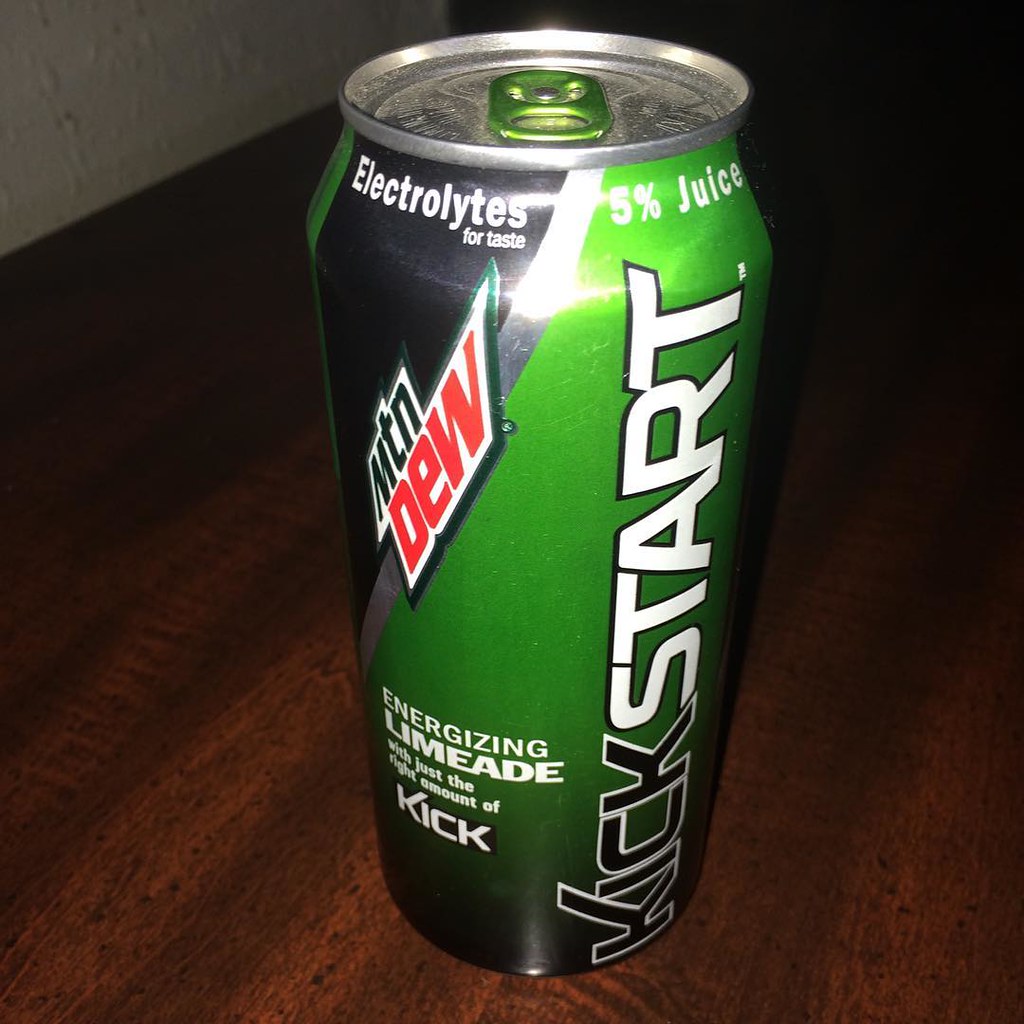This photograph captures a Mountain Dew energy drink can resting on a richly grained cherry wood table, accented by noticeable black wood grain patterns. In the background, a sliver of a white wall is visible, adding contrast to the scene. Natural light reflects off the sleek silver top of the can, highlighting its green pull tab. 

The can's design features the prominent Mountain Dew logo with "Mountain" abbreviated as "MTN" in a greenish hue, and "Dew" in a striking red. Below the brand name, the descriptive text appears: "kick" in black font, "start" in white font, and "energizing limeade" in white font, cleverly outlining the product's purpose.

Additional elements include a label stating "5% juice" in white font against a black background and "electrolytes for taste" also in white font. The light reflections on the can further emphasize its vibrant and crisp design, making it an eye-catching focal point against the naturally textured backdrop of the table.